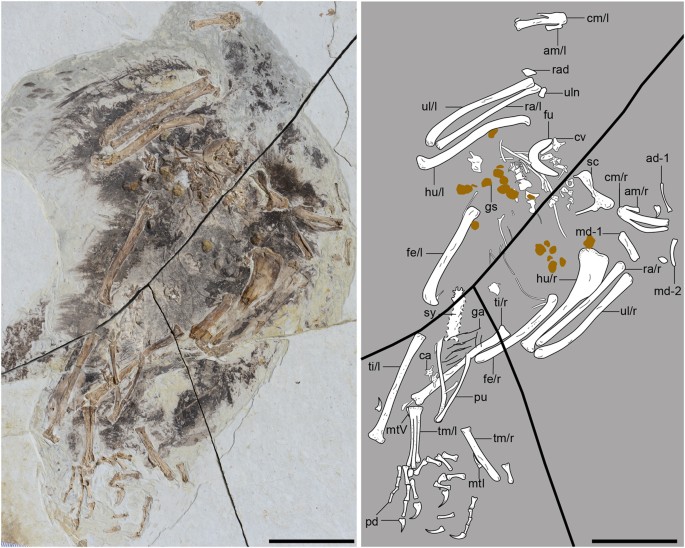The image consists of a side-by-side comparison. On the left side, there is a photograph depicting a flattened assembly of bones and feathers, likely the remains of a bird. The bones are jumbled together, creating a chaotic visual. On the right side, there is a detailed line drawing that systematically breaks down the same bones shown on the left. Each bone is individually portrayed and meticulously labeled, providing a clear and organized representation compared to the chaotic arrangement in the photograph. The line drawing enhances understanding by identifying specific bones and their placements within the skeletal structure of the bird.